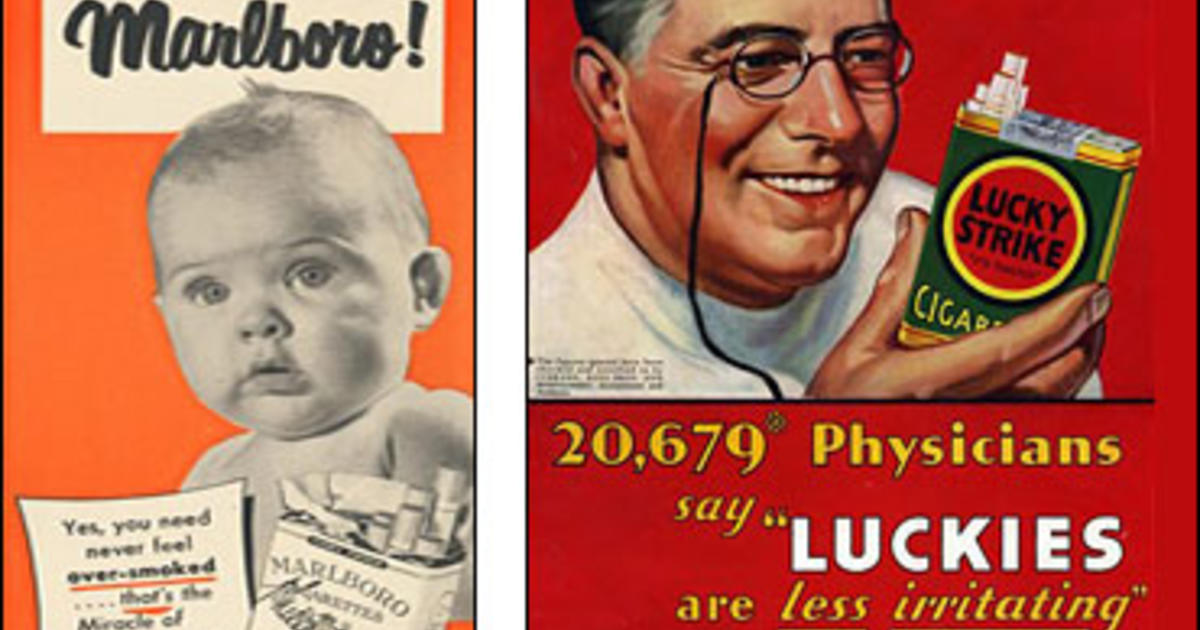The image features two juxtaposed vintage cigarette advertisements. The left poster, set against an orange background, depicts a black-and-white image of a wide-eyed baby. The text at the top of the poster, displayed in black cursive within an ivory-colored text box, reads "Marlboro!" At the bottom, another text box states, "Yes, you need never feel over smoked. That's the miracle of..." although the rest of the message is cut off. In front of the baby, there's a black-and-white pack of Marlboro cigarettes, with a few cigarettes poking out.

The right poster, which has a red background, showcases a prosperous-looking gentleman with gray hair, jolly red cheeks, and a monocle with a string attached. He is smiling and holding up a green pack of Lucky Strike cigarettes adorned with a red logo and yellow text. The pack similarly has a few cigarettes sticking out. Below this gentleman, the text in yellow asserts, "20,679 physicians say Luckies are less irritating." Both ads exhibit the striking and colorful design sensibilities of their era, making a bold statement side by side.